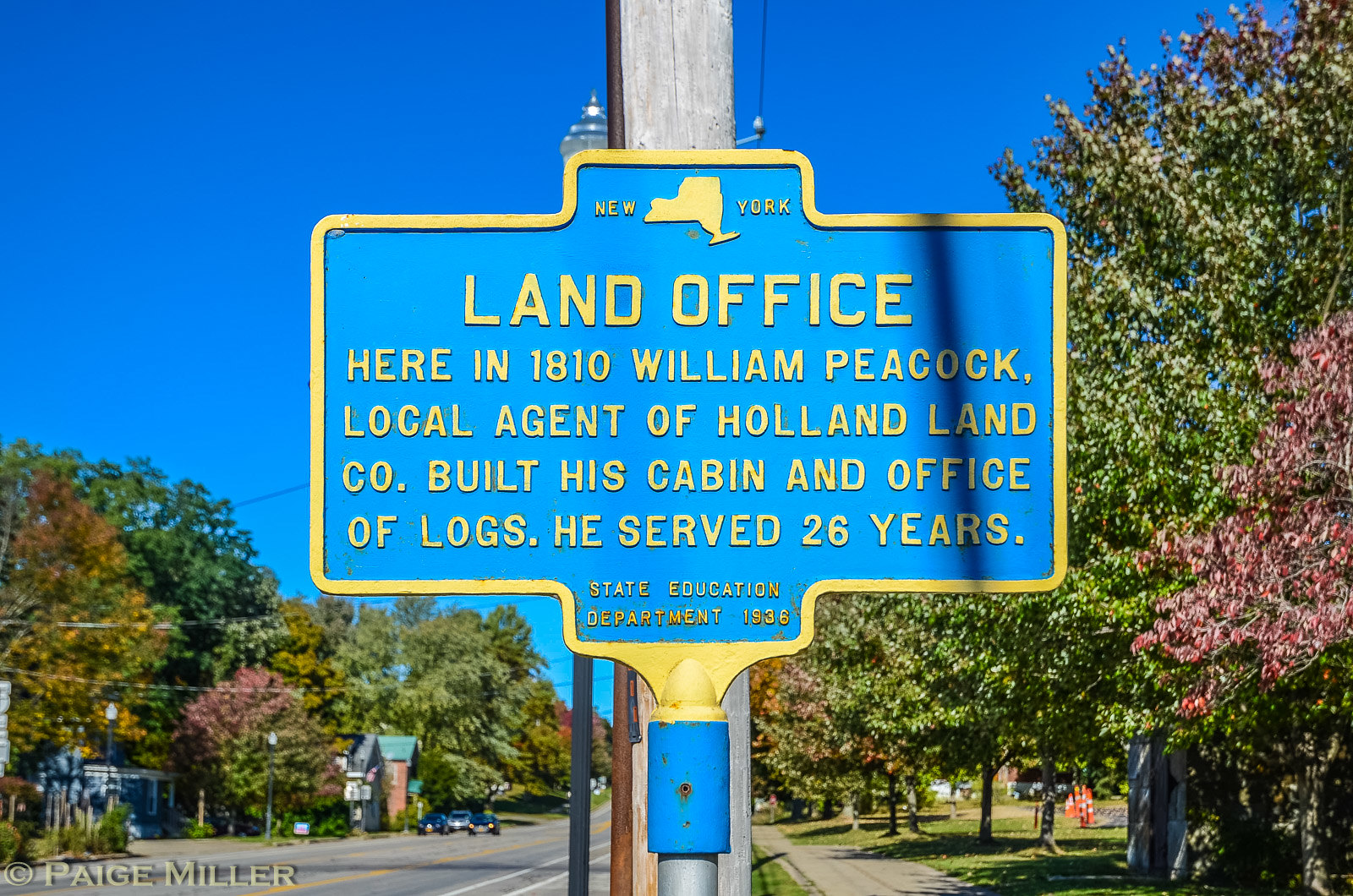This image depicts a vibrant street scene centered around an eye-catching historical sign. The blue and yellow sign, adorned with a rectangular shape featuring small protrusions at the top and bottom, is prominently displayed in front of a tall wooden post. The sign is meticulously detailed with yellow trim around its blue background and bold yellow text. At the top, it reads "New York" flanking a yellow silhouette of the state of New York. Beneath that, bold letters spell out "Land Office," followed by a historical note: "Here in 1810, William Peacock, local agent of Holland Land Co., built his cabin and office of logs. He served 26 years." At the bottom, in smaller text, it notes "State Education Department 1936."

The scene around the sign is picturesque, with a road stretching leftward into the distance and a sidewalk running parallel to it on the right. Both the road and sidewalk are lined with large trees showcasing leaves in vibrant shades of green, orange, and red, suggesting the photograph was taken in autumn. The sky is clear, a matching shade of blue to the sign, without a cloud in sight. Three vehicles are visible on the road, adding life to the serene setting. The photograph credits "Paige Miller" in the bottom left corner, presumably the photographer who captured this beautiful snapshot.